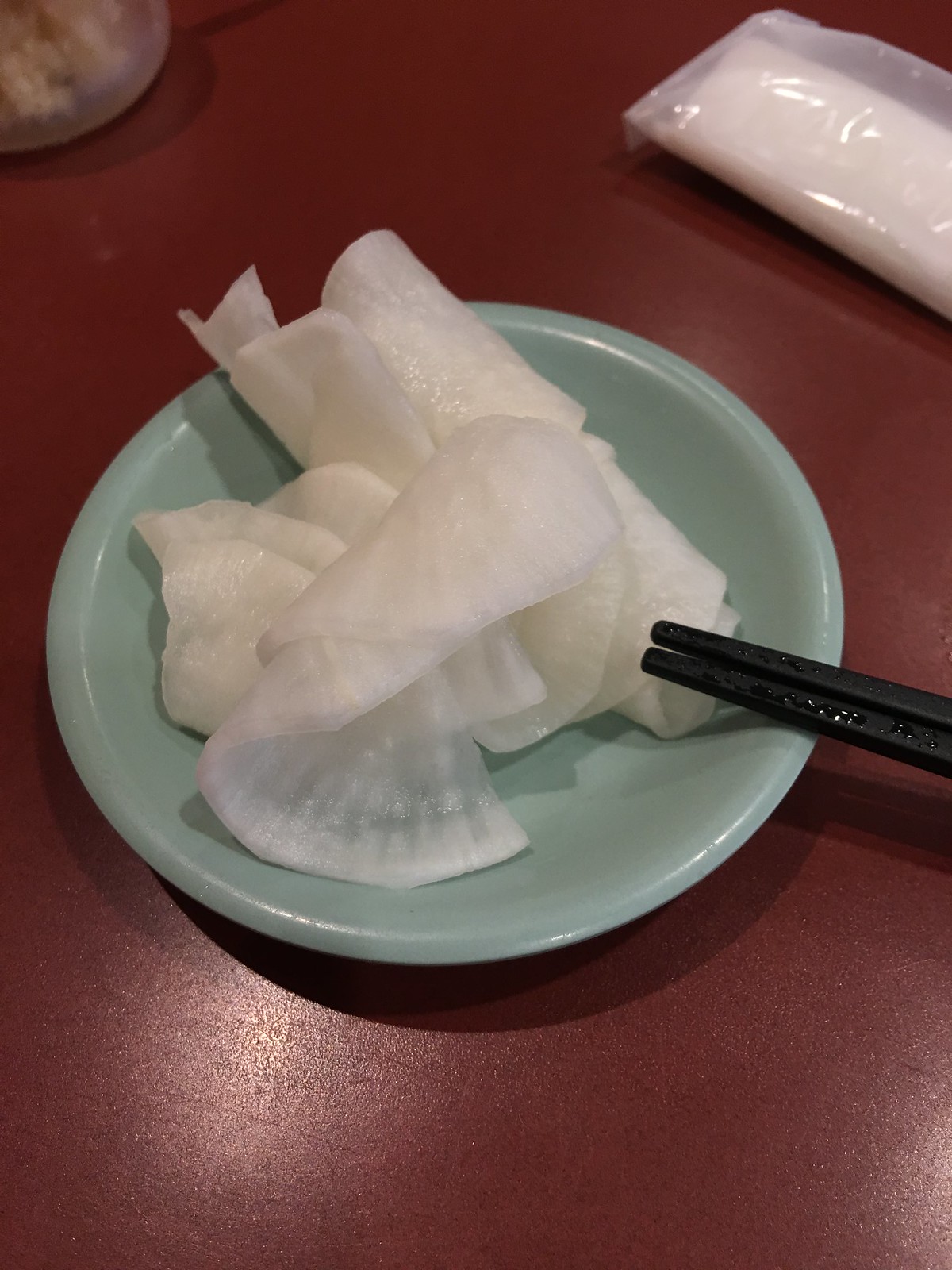The image showcases a meal with a prominent dish of glossy udon noodles, arranged artfully on a blue plate positioned at the center. The table underneath is a rich, deep reddish color, possibly maroon or copper-gray. Two sleek black chopsticks rest horizontally across the plate. In the background to the left, there's a white bag potentially containing more udon noodles, while the upper left corner of the image features either a bowl or container holding a gel-like substance, adding an element of intrigue to the scene. The meal is untouched, preserving its pristine presentation.